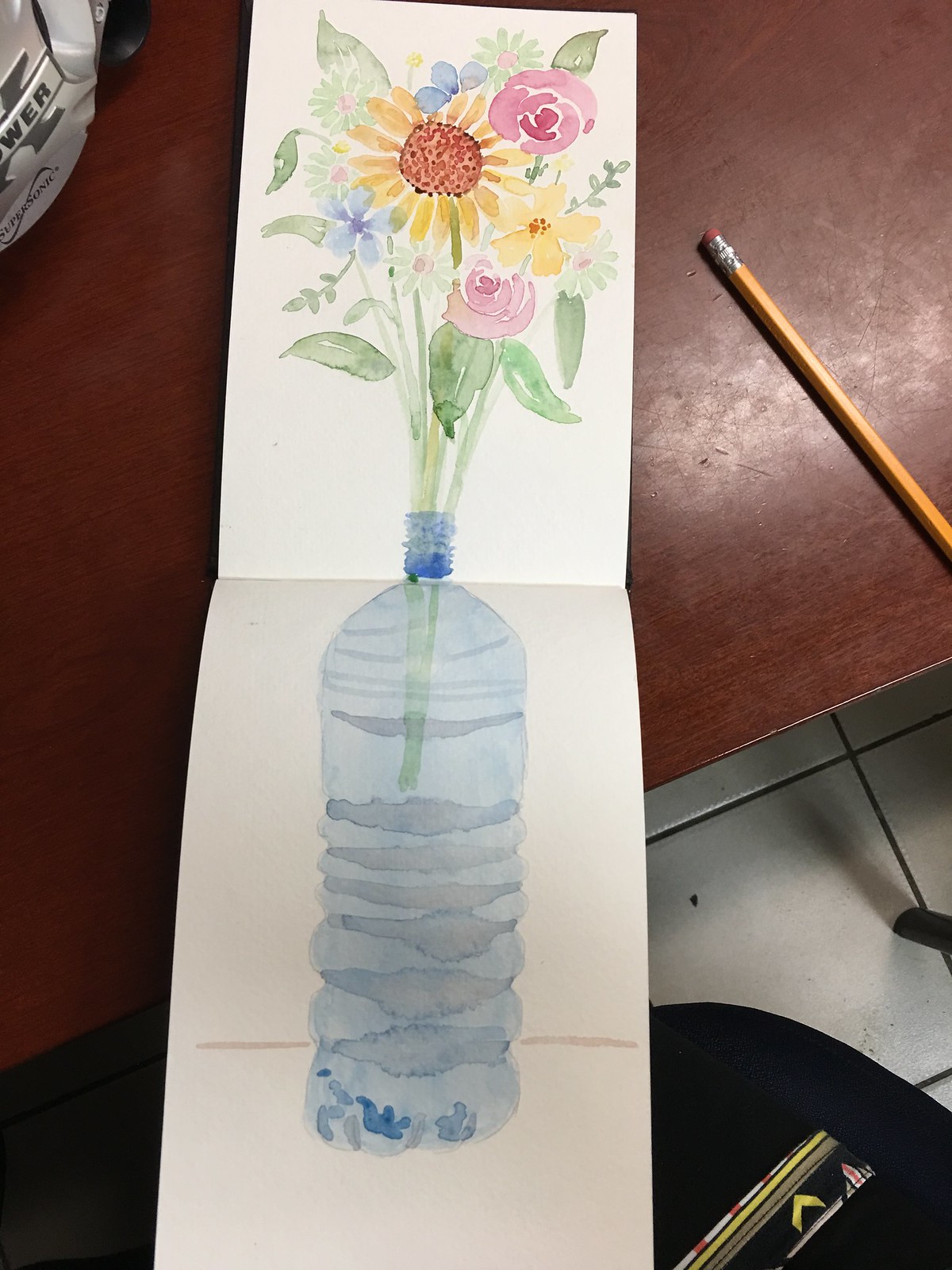This vertical image showcases a detailed watercolor painting on an art pad that is rectangular and vertically oriented. The artwork spans two open pages, depicting a vibrant bouquet of flowers arranged in a water bottle. The top page features the multicolored flowers, including yellow daisies, pink and red roses, and sporadic blue flowers with five petals. Surrounding the flowers are an abundance of lush green leaves. Some yellow flowers with five petals and orange centers add to the array of colors. The lower page reveals the water bottle, painted in a light pale blue with subtle purple shading. The entire arrangement is set atop a brown, wooden-topped table, providing a warm and natural backdrop to the exquisite floral composition.